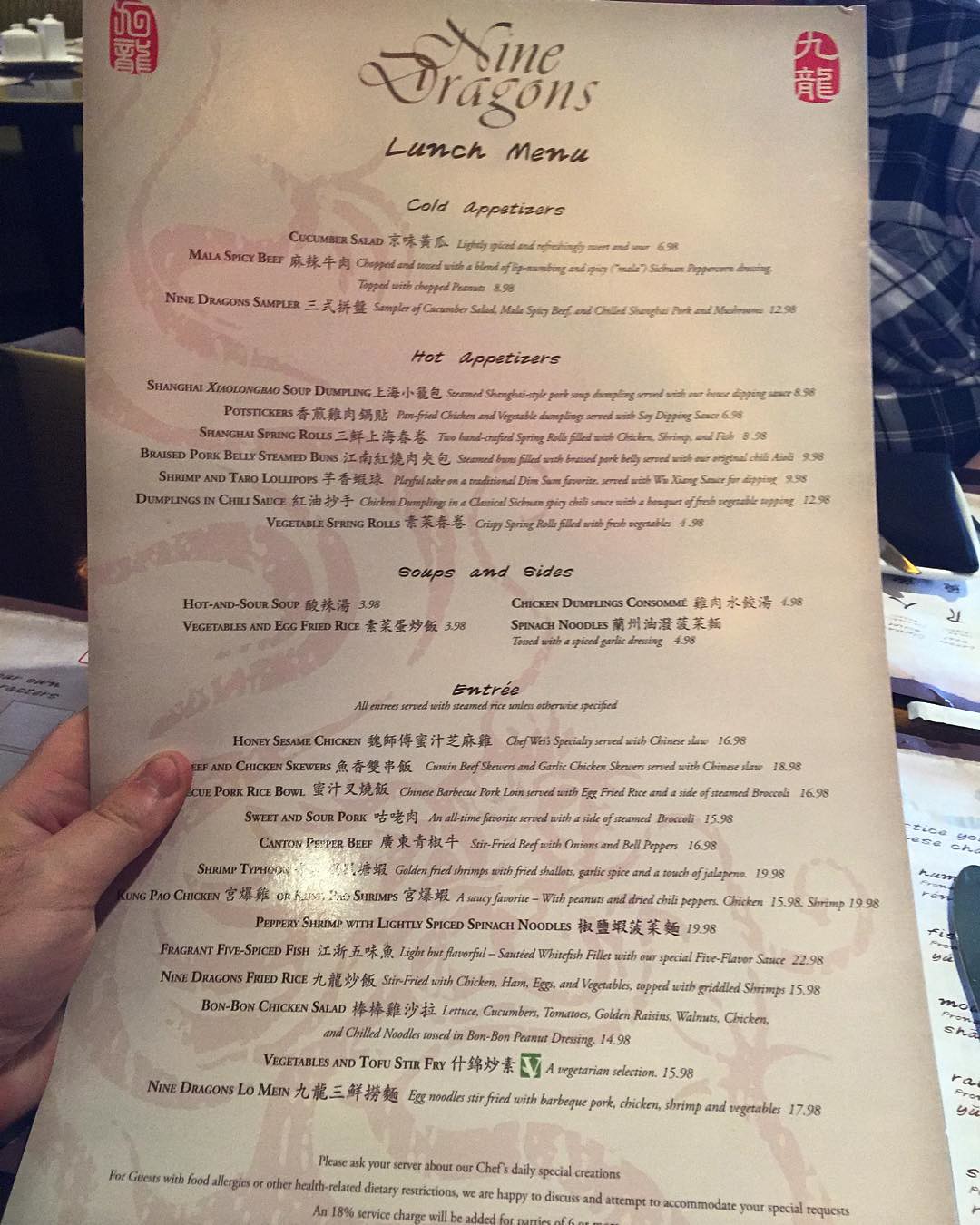In this photograph, a person is holding a large, off-white restaurant menu with their left hand. The individual's hand, which appears to belong to a white person, has short, untidy nails. The menu reveals intricate Asian-themed designs, including a background image reminiscent of a dragon. Titled "Nine Dragons," the menu specifies that it is for lunch and features sections for cold appetizers, hot appetizers, soups and sides, and entrees. The items are listed in both English and Chinese, with English descriptions accompanying each dish. In the upper corners of the menu, there are lantern-shaped red designs featuring Chinese characters.

Behind the menu, the person’s companion can be seen wearing a blue flannel shirt. To the left of this scene, another table is visible with white teapots on it, adding to the restaurant's ambiance. The detailed setting and cultural elements on the menu accentuate the Asian dining experience at Nine Dragons.